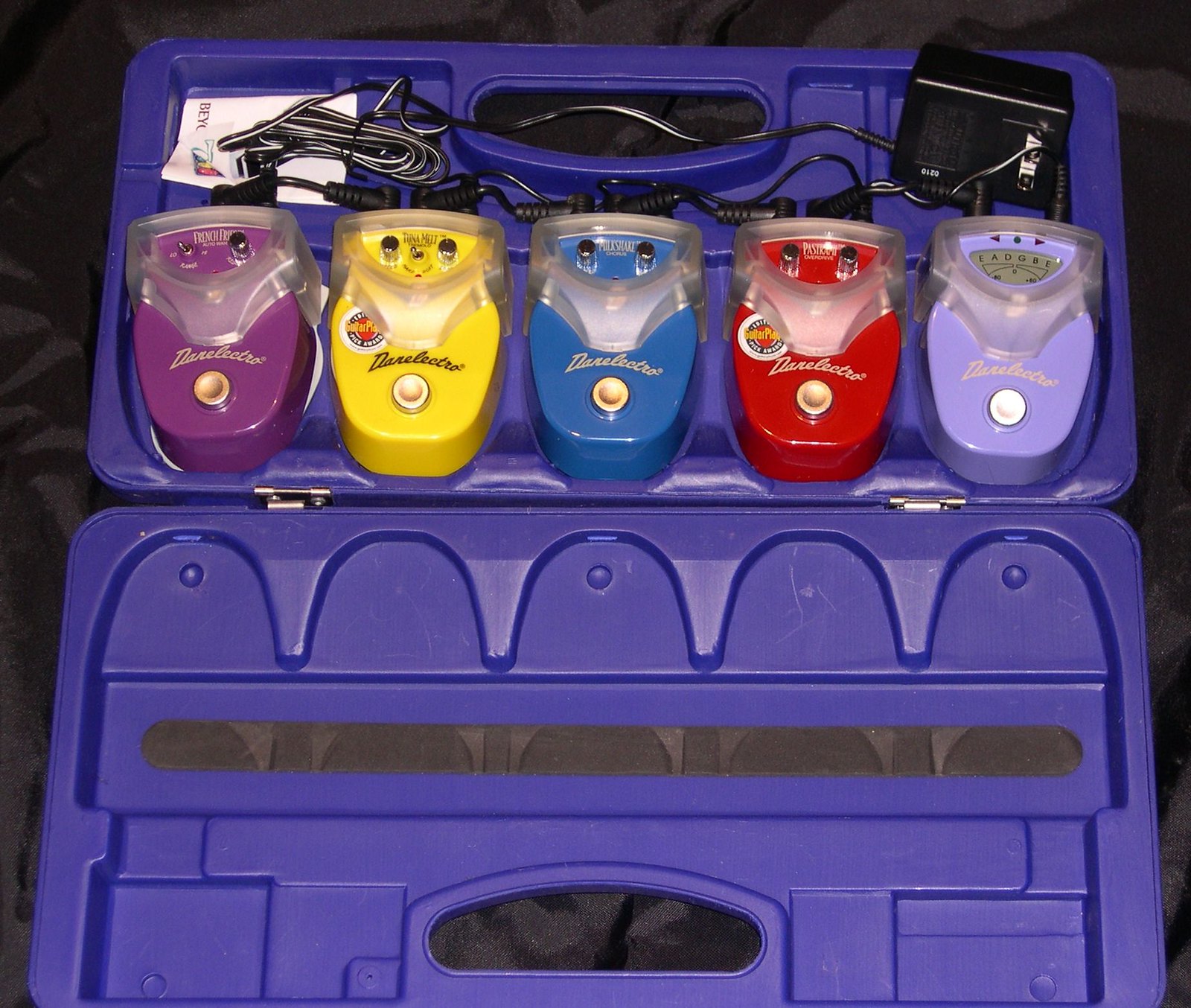The image depicts an open purple plastic travel case resting against a black and dark gray background. Inside, the case reveals five colorful guitar pedals arranged from left to right in purple, yellow, blue, red, and lavender. Each pedal, made of shiny, enamel-painted metal, features a central foot switch for activation. The pedals also display various knobs and switches at their tops, with the lavender one uniquely equipped with an LCD screen. The visible logo on the pedals is curved and in a scripted font, reading "Dare Electro." Additionally, black electrical cords, a charger, and a clear foot shield to prevent accidental adjustments are visible, highlighting the pedals’ adaptability for different electrical setups.